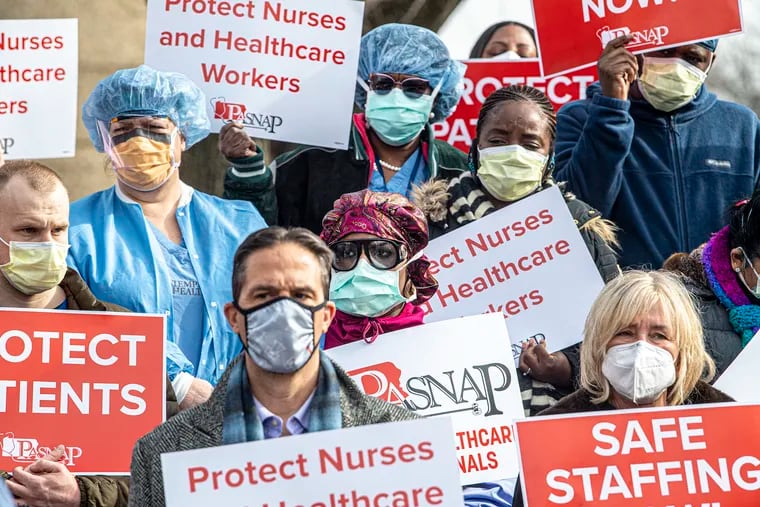In this powerful and emotive image, a diverse group of protestors is captured standing together at what appears to be a demonstration advocating for healthcare workers. Each individual is wearing a face mask, adhering to safety protocols. 

In the foreground, two protestors stand side-by-side. On the left, a man donning a cloth face mask holds a white sign with bold red lettering that reads "Protect Nurses," though the bottom portion of the sign is cut off. Next to him is a woman with blonde hair, wearing a white N95-style face mask. She clutches a red sign with white text stating "Safe Staffing," with its lower part also cropped out of the frame.

Just behind and above them, another cluster of individuals can be seen. An African-American woman dressed in a pink outfit and hat, wearing black goggle-like glasses and a light green surgical mask, holds a white sign that reads "PA Snap," though part of her sign is similarly obscured. Beside her stands a man in a brown coat; he holds a red sign with partially obscured white writing and wears a yellow surgical mask.

In the next tier of individuals, a woman is clad in a blue surgical gown, matching surgical bonnet, face mask, and face shield. Next to her, another African-American woman with braided hair wears a yellow face mask that reads, "Protect Nurses and Healthcare Workers."

At the top, another African-American woman, wearing sunglasses and a surgical bonnet, holds a sign with the same wording, "Protect Nurses and Healthcare Workers."

This image vividly depicts the solidarity and determination of a diverse group of individuals, united in their advocacy for better conditions and protections for nurses and healthcare workers.